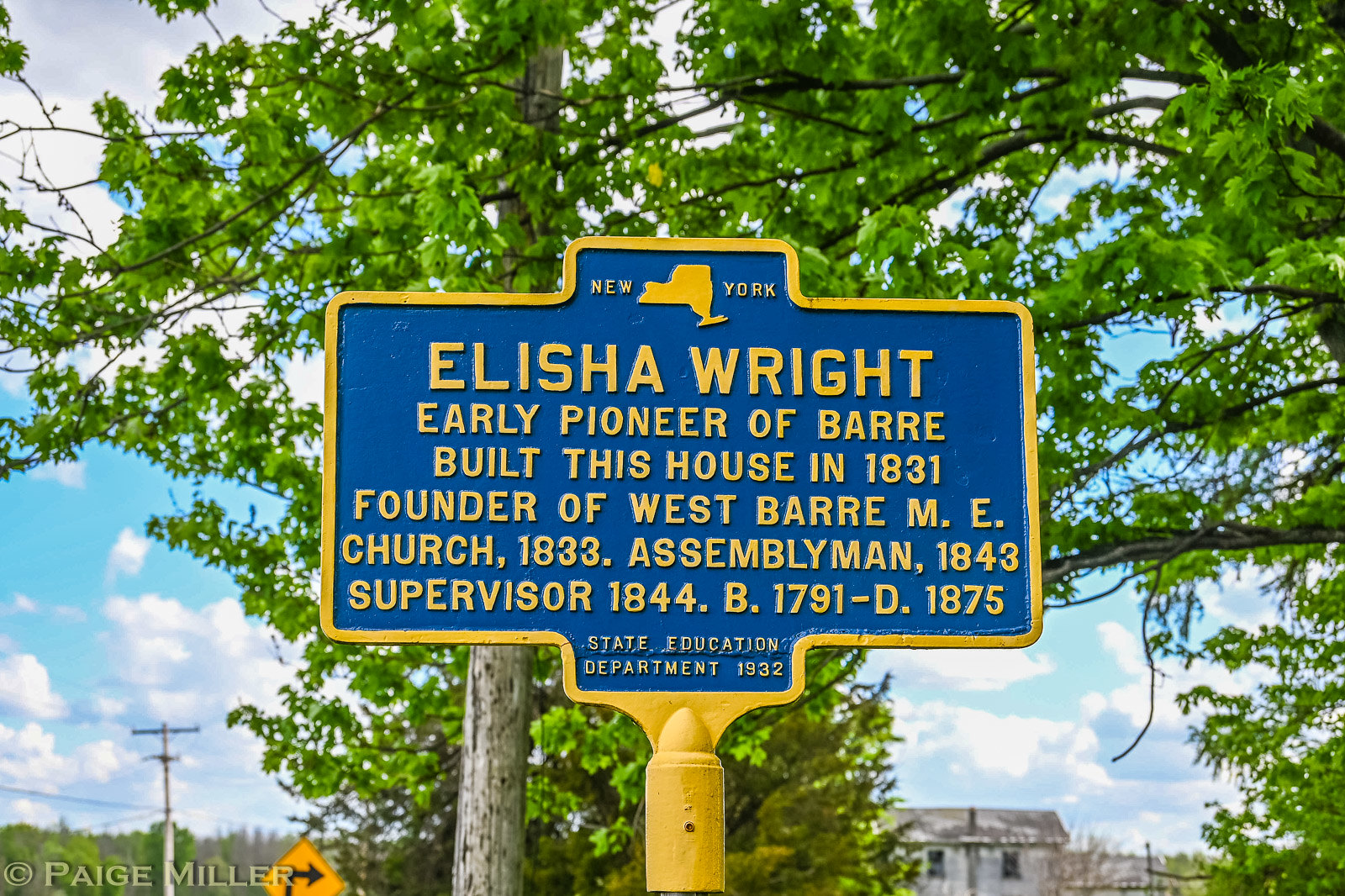The photograph depicts a blue and yellow historical marker sign with the following detailed description. The metal sign features a yellow border and post, and has raised yellow text on a blue background. The top of the sign displays the outline of the New York state map and the word "New York." Below, in bold capital letters, it reads "Elisha Wright," followed by smaller capital letters detailing his accomplishments: "Early pioneer of Barre, built this house in 1831. Founder of West Barre M.E. Church, 1833. Assemblyman, 1843. Supervisor, 1844." Additional information includes his birth and death years, "B. 1791 - D. 1875," and the sign's establishment date, "State Education Department, 1932." The background reveals a residential area with trees, a power pole or tree trunk, and a distant, slightly blurry old house. The lower left corner of the image contains a watermark stating "Copyright Paige Miller."